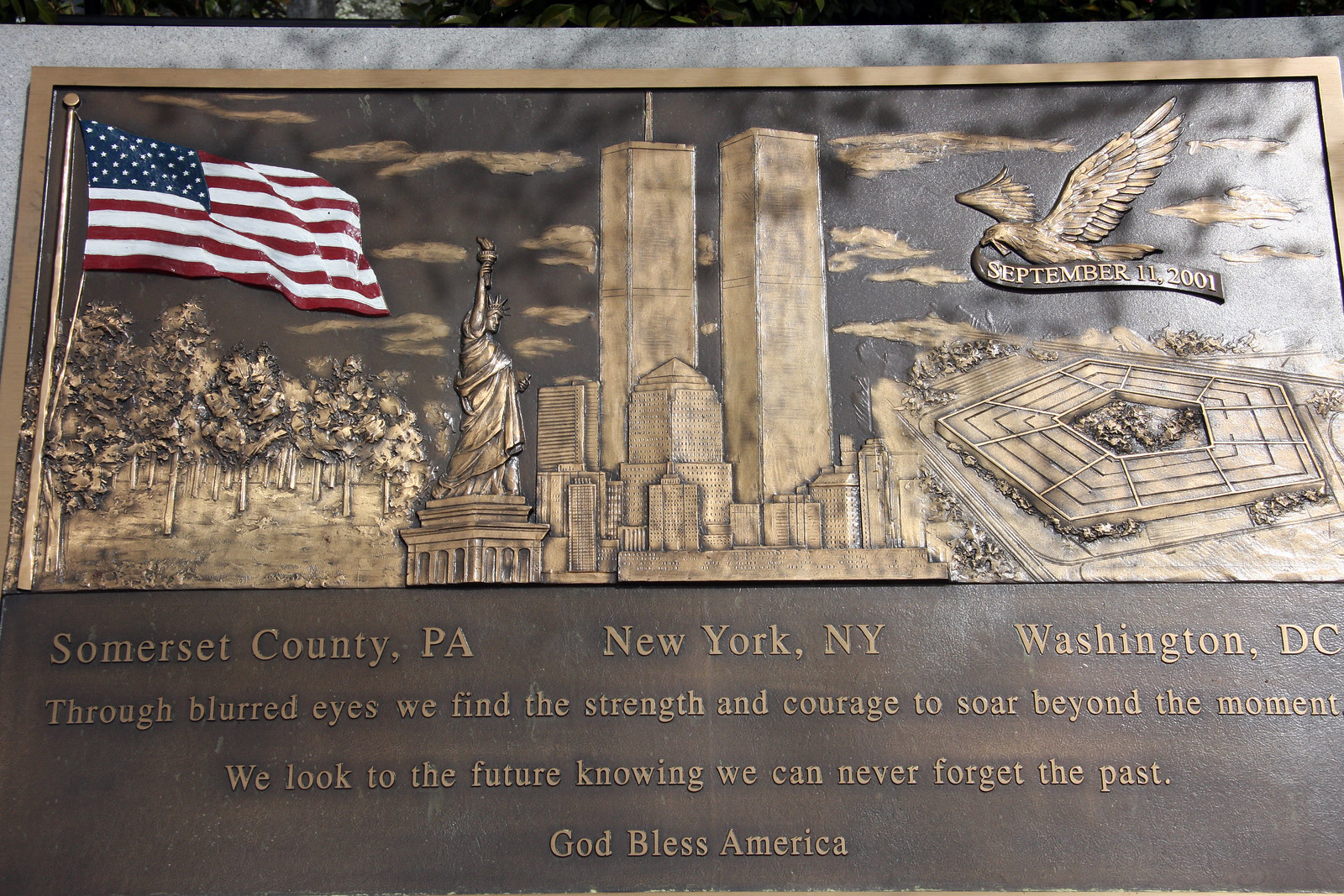This detailed metal plaque, possibly made of bronze or a golden-colored hard material, serves as a poignant memorial for September 11th, 2001. The plaque features a bas-relief depiction of the Twin Towers, the Pentagon, and the Statue of Liberty. An American flag is etched to the left, while an eagle carries a ribbon in its beak bearing the date, September 11, 2001. Additional imagery includes trees, clouds, and cityscapes. Inscribed on the plaque are the locations Somerset County, Pennsylvania, New York, New York, and Washington, D.C., alongside the quote: "Through blurred eyes, we find the strength and courage to soar beyond the moment. We look to the future knowing we can never forget the past." The bottom of the plaque proclaims "God Bless America." It measures approximately a foot and a half by a foot and appears to be placed on a marble countertop or mounted on concrete, possibly at a memorial site.